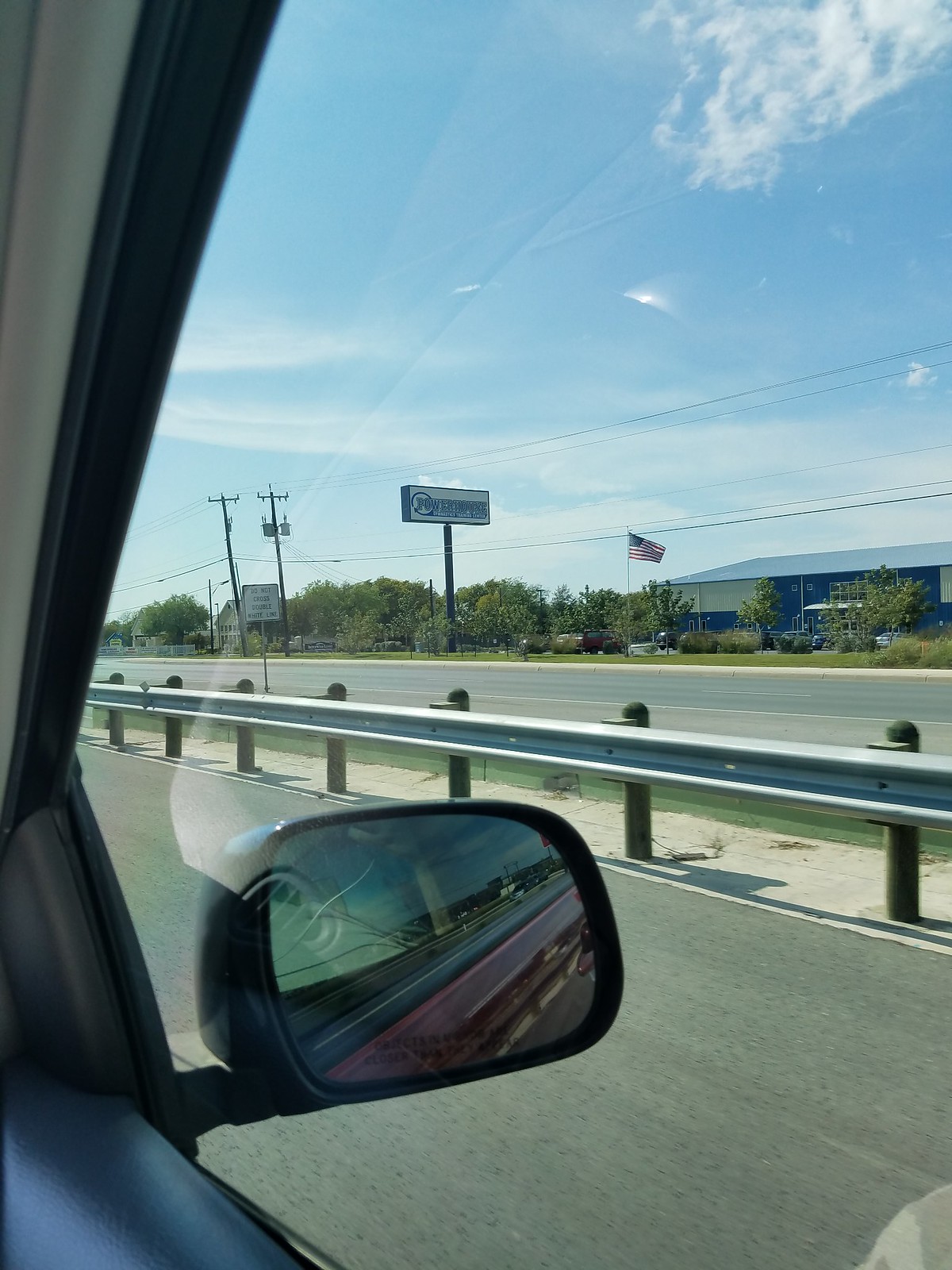The photograph captures a scene from the passenger side of a vehicle traveling on a highway. The frame of the car's window is partially visible, along with a reflection in the glass. Prominently featured is the side mirror, which reveals part of the vehicle's surroundings. The highway's asphalt surface is clearly seen, bordered by a gray metal guardrail. Beyond the guardrail lies another stretch of highway. In the distance, a tall sign mounted on a large metal pole stands out, though the blue lettering on the rectangular sign is not legible due to the distance. This sign is associated with a blue building that can be seen further away, forming part of the backdrop of the scene.